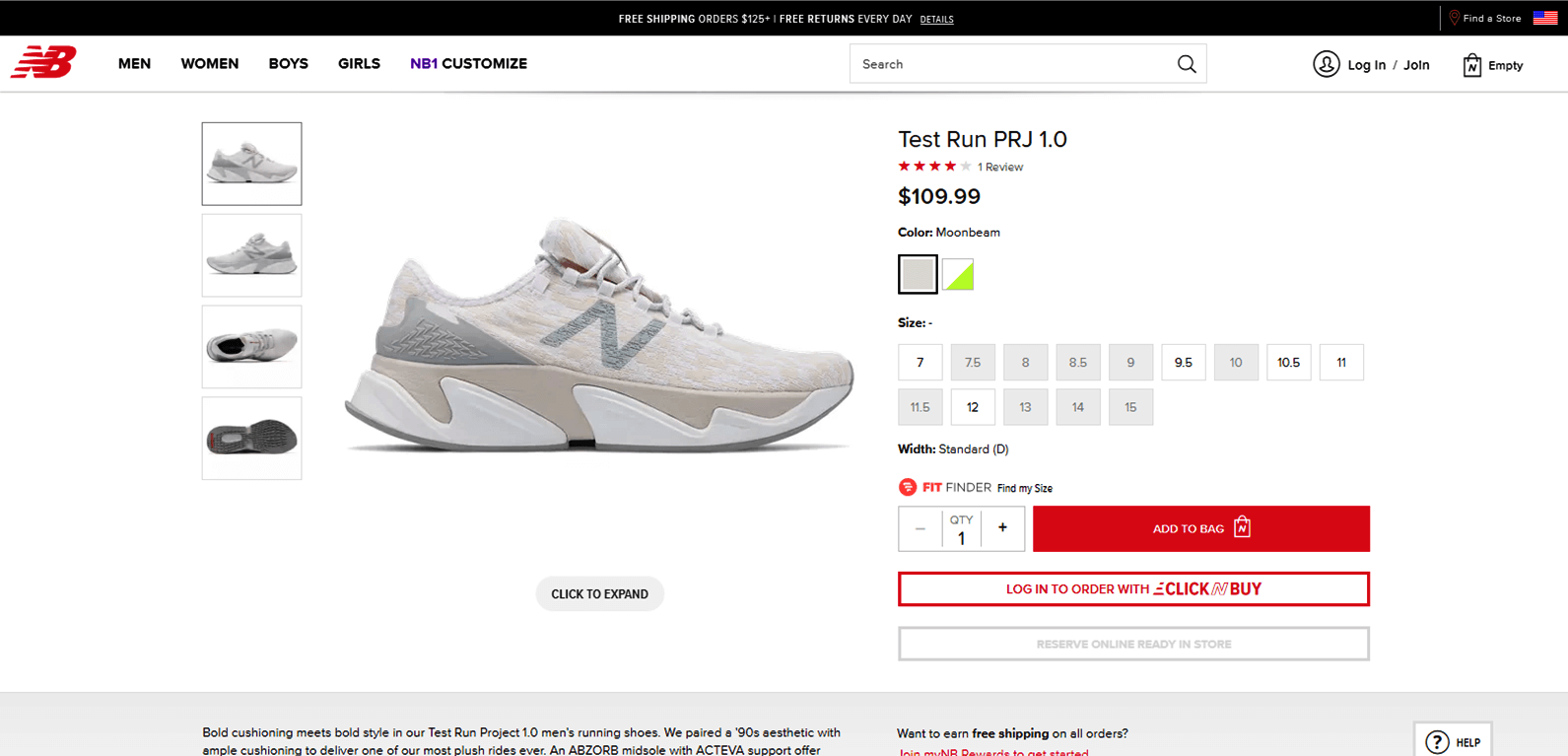This is a detailed screenshot of the New Balance website featuring the Test Run PRJ 1.0 sneaker. At the very top, a black promotional bar highlights offers like "Free Shipping on Orders $125+" and "Free Returns Every Day," with a clickable "Details" link. On the right end of this bar, there's a "Find a Store" text in white, accompanied by an American flag icon.

Below this bar, another navigational strip showcases the New Balance logo in red, followed by menu options: Men, Women, Boys, Girls, NB1 Customize, a search bar, a "Login/Join" section featuring a circle with an avatar icon, and a shopping bag icon marked with an "N" indicating the cart is empty.

Front and center is the product presentation for the Test Run PRJ 1.0 sneaker. The main image displays the shoe with light shades of gray and tan, featuring a wave pattern along the heel and bottom. Four thumbnail images provide different angles of the shoe, with the topmost thumbnail currently selected. The displayed color option is "Moonbeam."

Sizing options are clearly visible, with the available sizes being 7, 9.5, 10.5, 11, and 12. Sizes 7.5, 8, 8.5, 9, 10, 11.5, 13, 14, and 15 appear grayed out, indicating they are unavailable. The selected width is "D Standard." A "Fit Finder - Find My Size" icon is located below the sizing options, likely to assist customers in selecting the right size.

To the right of the sizing options, a quantity selector allows the user to adjust the purchase quantity with minus and plus buttons enclosed in rectangular boxes. Next to this, an "Add to Bag" action button is prominently displayed. Further down, a "Login to Order with Click & Buy" option appears, with "Click & Buy" being emphasized as a brand offering. A grayed-out "Reserve Online in Store" button is also visible.

At the bottom of the page, a gray box contains fine print text providing additional details about the sneaker.